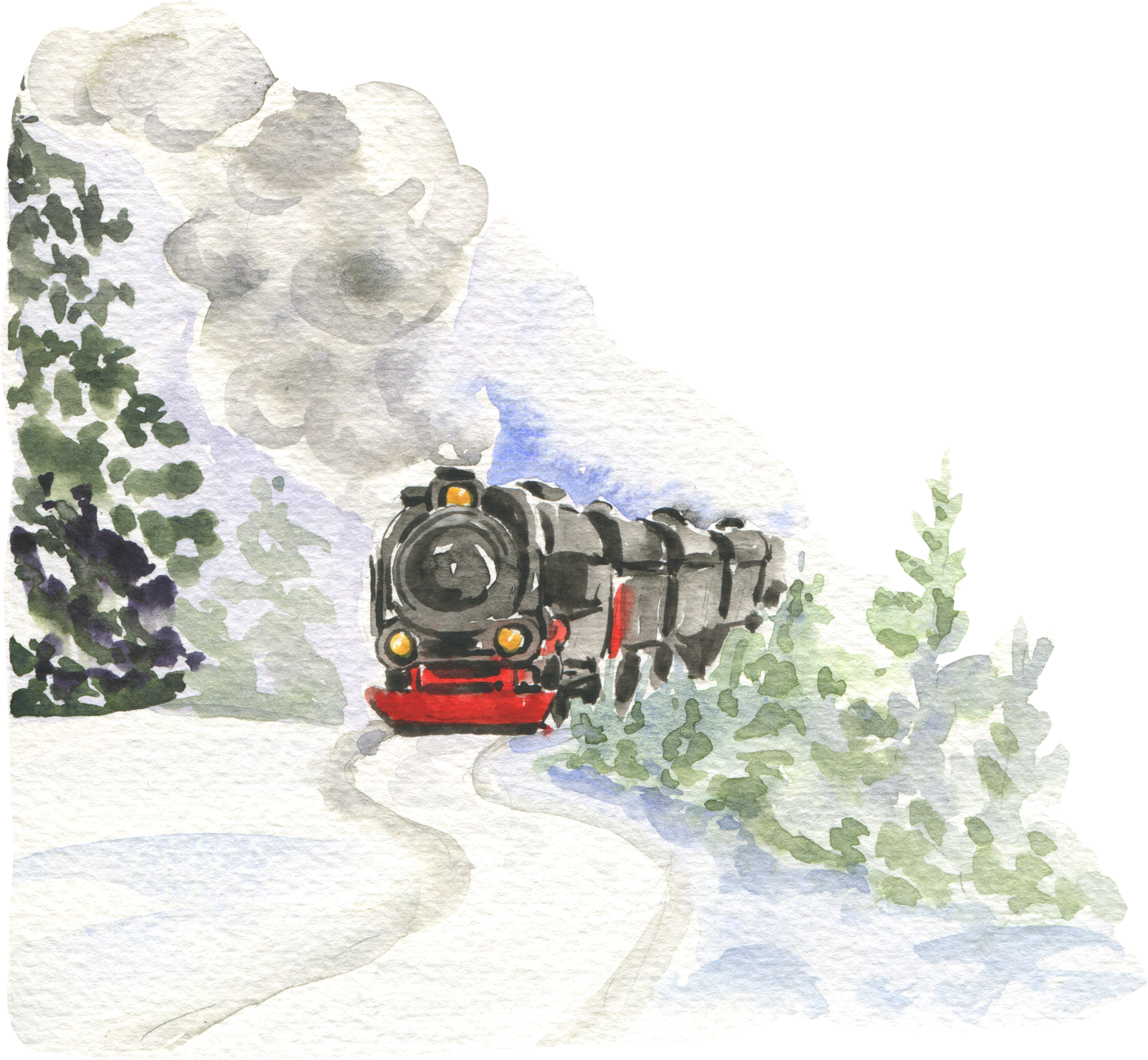The watercolor painting depicts an old-fashioned steam locomotive chugging towards us on snowy tracks, winding their way through a wintry landscape. The impressionistic style makes the scene slightly less defined, but details emerge clearly: the locomotive is black with red on the bottom and three glowing yellow lights adorning the front. Puffy clouds of black, gray, and white smoke billow from its smokestack. To the left, a tree with a mix of green and black hues stands among other green and gray foliage. The foreground showcases the snow-covered tracks, while the background reveals hints of a blue sky. The train, pulling three cars behind it, embodies a journey through a serene, snow-laden setting, captured beautifully in watercolor strokes.